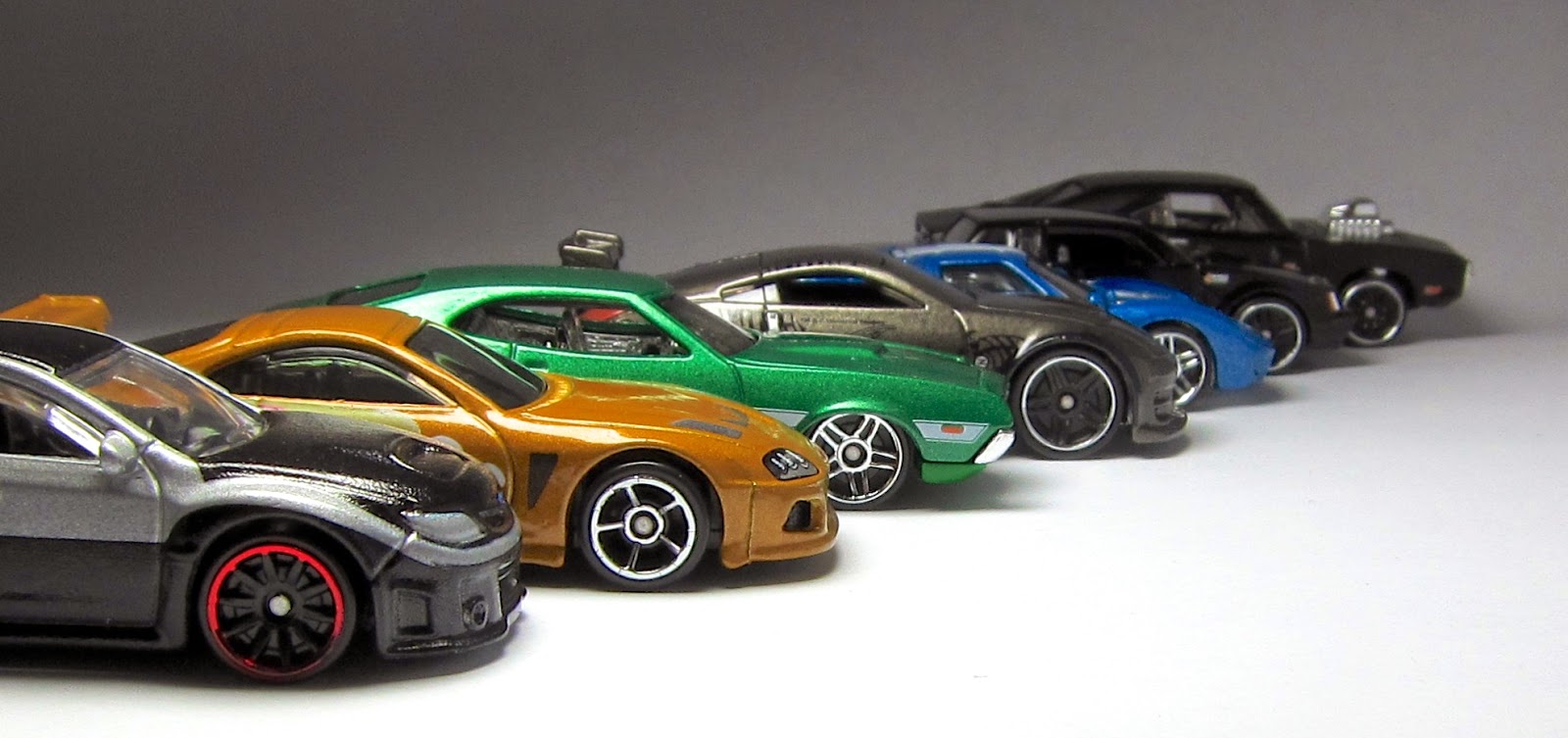This image features a lineup of seven die-cast toy cars, reminiscent of classic Matchbox or Hot Wheels from the 1970s to the 1990s, arrayed diagonally from the bottom left to the top right. The cars range in color and model, with the furthest being a black 1960s muscle car, possibly a Camaro with a chrome engine blower. Next to it is another black car, likely an '86 Grand National. The third car in line is a blue Ferrari model, followed by a silver Nissan 350Z. The fifth car in the sequence is a green Plymouth Charger, then a yellow-orange vehicle, potentially a Toyota Supra, and finally, the closest car is another Toyota Supra, featuring two shades of gray. Each car's right wheel is at least partially visible. The background is plain and entirely white, suggesting a nondescript or warehouse setting.